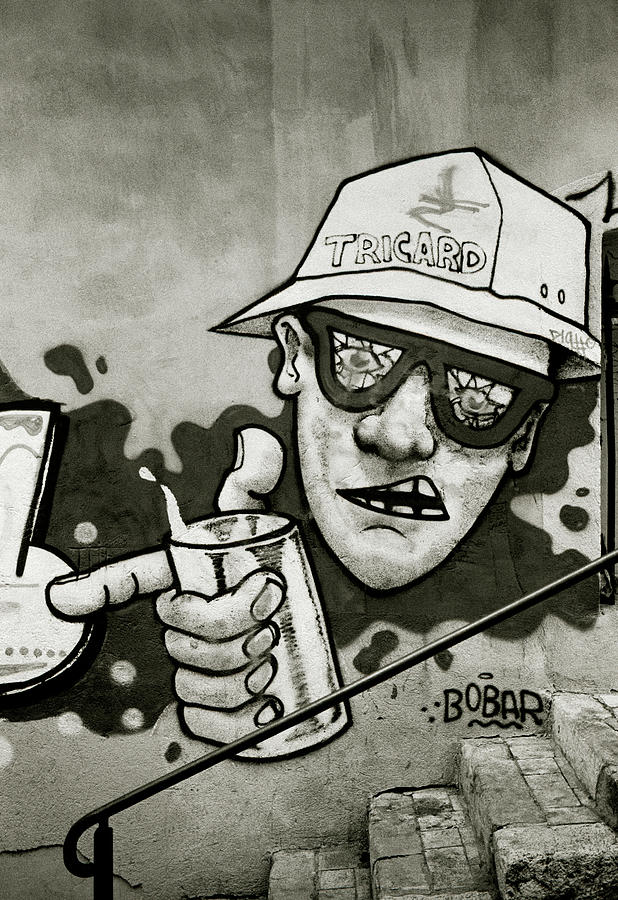The image displays a highly detailed black, white, and gray street art scene done in a style reminiscent of abstract graffiti or a comic panel. The central figure is a male character wearing a cap labeled "Tricard" and a pair of broken glasses, with his mouth open as if caught mid-expression. Distinctively, he has six fingers gripping a can of drink, with liquid splashing out from the top. The background features various shapes and shading, including a staircase with a metal handrail at the bottom. Graffiti text stating "Bobar" underlines the man's face, which is oriented towards the viewer, conveying a direct and dynamic interaction. The piece, signed by the artist Bobar, includes elements that blend seamlessly into its inked background, leaving some parts intentionally ambiguous. The overall composition suggests a professional yet edgy execution typical of urban wall art.